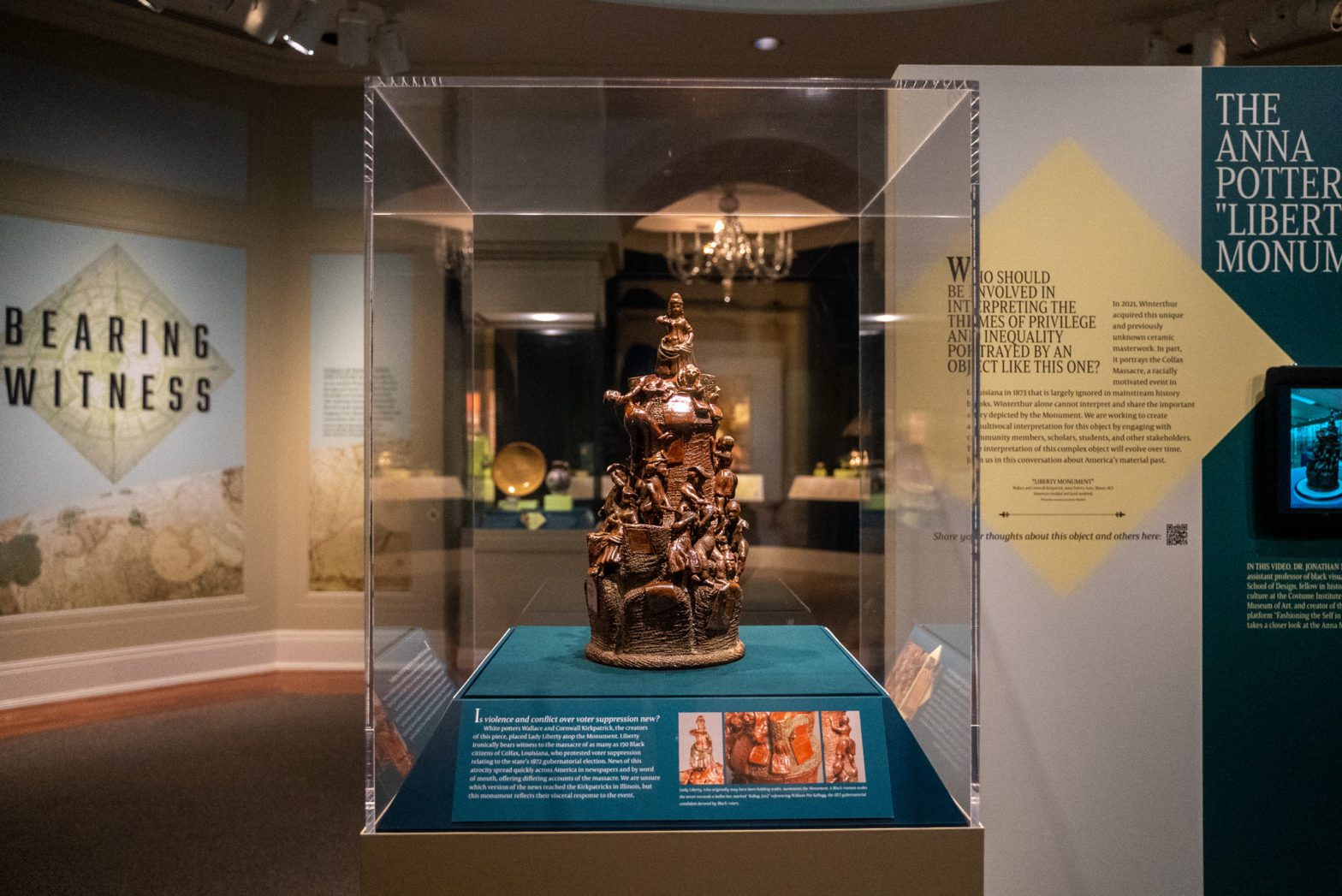The image showcases a detailed, hand-carved ceramic masterwork titled the Anna Potter Liberty Monument, encapsulated in a glass case. The sculpture, part of the museum's Bearing Witness program, represents an unreported incident in African-American history, specifically the Colfax Massacre of 1872 in Louisiana, which occurred following protests against voter suppression. At the top, a depiction of Lady Liberty or possibly a seated Buddha is prominently featured above smaller figures that appear to be struggling or climbing. The piece, recognized as a unique and previously unknown ceramic masterwork created by two white sculptors, vividly interprets themes of privilege and inequality. Surrounding the display are posters, with one prominently reading "Bearing Witness," enriching the narrative context of the artwork. Other inscriptions on the display are difficult to read, adding an element of mystery to the comprehensive interpretation of this significant piece.